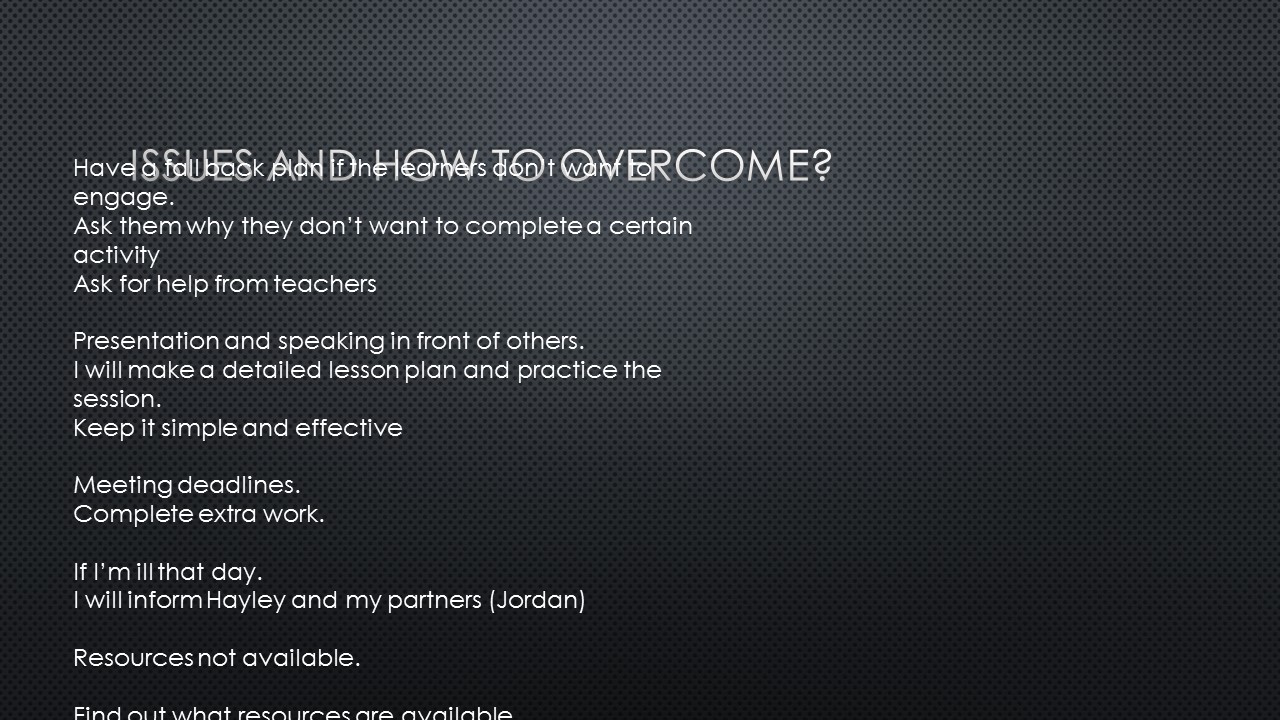The image features a gray-black background with dotted patterns, overlaid with white text. The title, "Issues and How to Overcome?" is prominently displayed at the top left, though it partially overlaps with the initial lines of the subsequent text. The text that follows offers strategies for addressing various classroom challenges. It suggests having a fallback plan if learners are disengaged, asking them why they resist completing activities, and seeking help from teachers. The text also covers the importance of presentations and public speaking, recommending the creation and practice of detailed lesson plans. It emphasizes keeping sessions simple and effective, meeting deadlines, and completing additional work. There is also a note about informing Haley and a partner if ill, with a bracketed comment about unavailable resources followed by advice to identify available ones. All text appears in small white letters against the dark background, creating a contrast that highlights the instructional content.